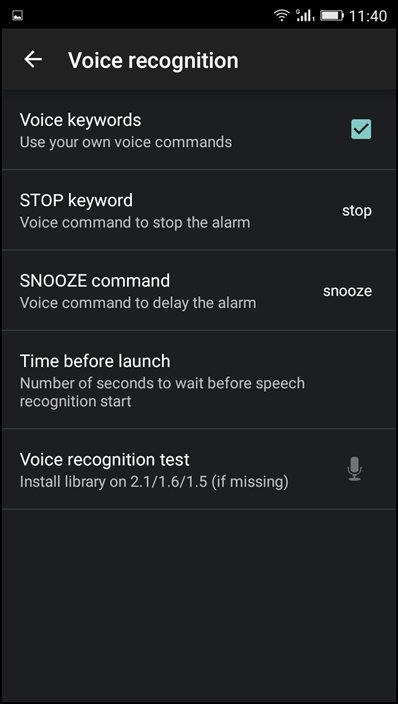The image displays a mobile device screen within the Voice Recognition section of its settings. At the top of the screen, a thin black border holds a notification from the Photos app in the upper-left corner. Adjacent to it on the right, there are icons for Wi-Fi, cellular signal, battery life, and the current time, which is 11:40.

Below the black border, there's a gray header featuring a white back arrow and the text "Voice Recognition" in bold white letters. The following section has a darker gray background with various options listed:

1. **Voice Keywords** - "Use your own voice commands" is indicated with a checkmark next to it, signifying that it is enabled.
2. **Stop Keyword** - "Voice command to stop the alarm," listed as "Stop."
3. **Snooze Command** - "Voice command to delay the alarm," listed as "Snooze."
4. **Time Before Launch** - Specifies the "Number of seconds to wait before speech recognition starts."
5. **Voice Recognition Test** - Notes the installation for libraries on versions 2-2.1, 1.6, and 1.5 if missing.

Each of these settings is clearly listed to ensure users can customize their voice recognition preferences easily.